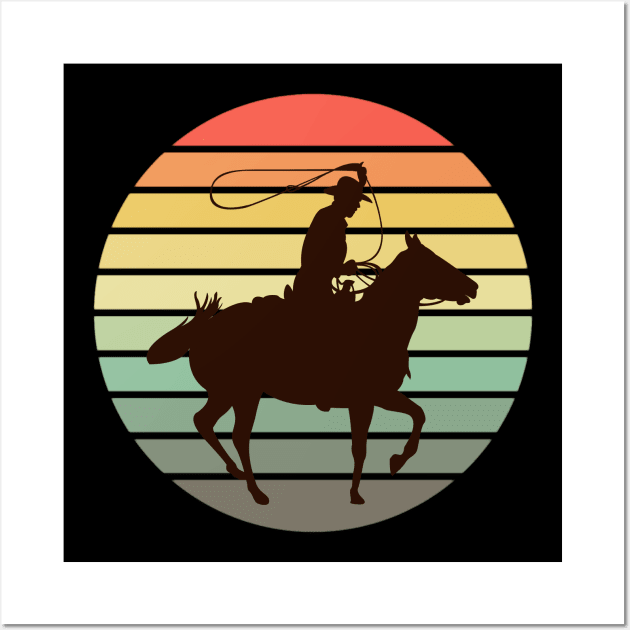The image depicts a striking, minimalistic graphic design set on a square piece of white paper, resembling the format of a greeting card. Encased in a clean white border, the main feature of the image is a square black background with a centrally positioned circle that almost extends to the edges. This circle is artistically divided into about ten horizontal stripes, transitioning through various colors — from a reddish tone at the top, through shades of orange, goldenrod, yellow turning into pale green, and gradations of turquoise, down to slate and gray at the bottom where the horse's hooves are positioned.

At the center of this colorful circle is a detailed silhouette of a cowboy on a dynamically posed horse, both in mid-motion. The horse, shown in profile facing right, has its right front and rear legs lifted, adding a sense of movement. The cowboy, clad in a traditional hat, has his left hand raised, skillfully twirling a lasso above his head, while the rest of the rope is held in his right hand just above the saddle. The horse's tail is captured swishing to the side, enhancing the dynamic feel of the scene. This evocative silhouette, with its crisp black lines, contrasts starkly against the vibrant stripes, making for a striking visual representation of Western life.